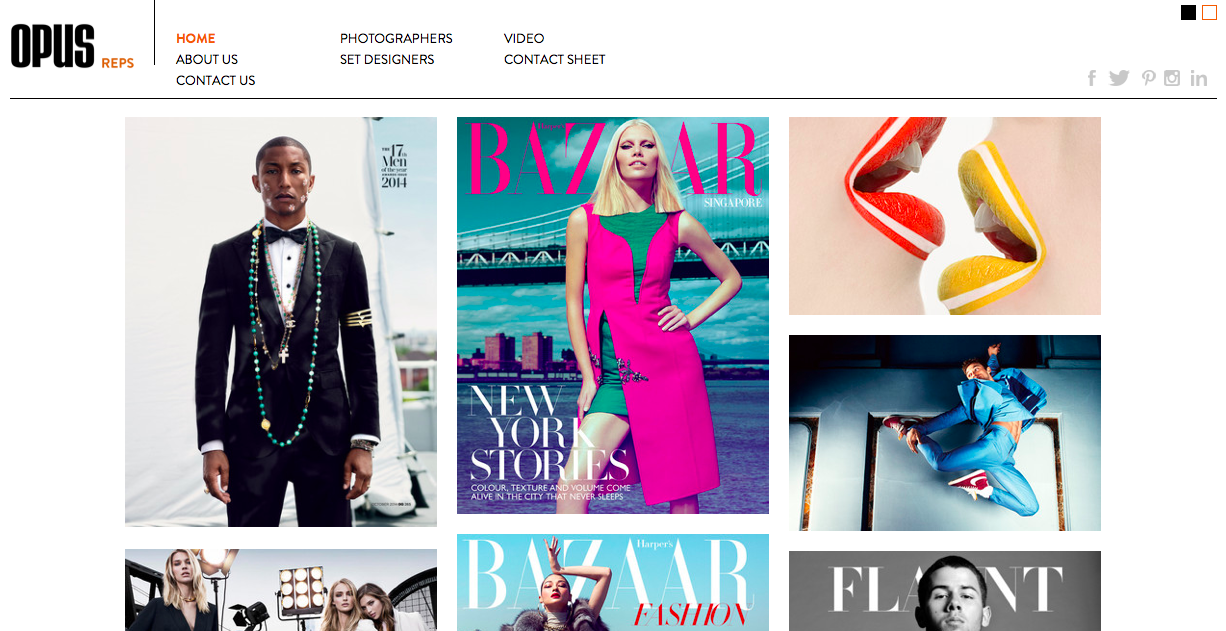Screenshot of the Opus Reps Website

In the screenshot of the Opus Reps website, the branding and layout elements are clearly visible. In the top left corner, the name "Opus Reps" is displayed, with "Opus" in bold, large, black font, while "Reps" is smaller and in an orange color. Adjacent to the name are several navigation categories, including Home, About Us, Contact Us, Photographer, Set Designers, Video, and Contact Sheet. The Home category is highlighted in orange, indicating the current active page, while the other categories are in black font. 

On the top right, a series of sharing options can be seen, likely for Facebook, Twitter, Pinterest, Instagram, and LinkedIn, represented by the abbreviation "IN."

The central focus of the site is a collection of various magazine covers featuring prominent celebrities and striking photographs. 

- **Top Left:** Pharrell Williams, adorned with multiple necklaces and wearing a tuxedo, is depicted with flowers on his face, seemingly outdoors.
  
- **Middle:** The cover of Bizarre Singapore showcases a blonde woman posing with her hand on her hip (right side for viewers). She is donning a pink and green dress, with the Brooklyn Bridge in the background, and the cover headline reads "New York Stories."

- **Adjacent to Pharrell's Image:**
   - **Top Smaller Photo:** Two individuals' lips are prominently displayed. One on the left has predominantly red lips with a white stripe, while the right one has mostly yellow lips with a white stripe.
   - **Below the Smaller Photo:** A man is captured mid-air, striking a pose with his feet turned to his right (viewer's left). He is clad in a blue three-piece suit, exuding motion and style.

- **Bottom Row (Partial Images):**
   - The bottom left image shows three women, two blondes and one brunette (on the right), in a studio surrounded by bright filming lights and equipment.
   - The center image features a woman with her hair pulled back or shaved, her left hand resting on her head in a pose. The overlay reads "Harper's Bizarre Fashion," and she's partially clad in what appears to be a fur vest or jacket.
   - The bottom right corner reveals part of Nick Jonas's face, with his head partially obstructing the word "Flaunt." The image is rendered in black and white.

This detailed collection of imagery and the structured interface highlight the vibrant and eclectic range of content offered by the Opus Reps website.